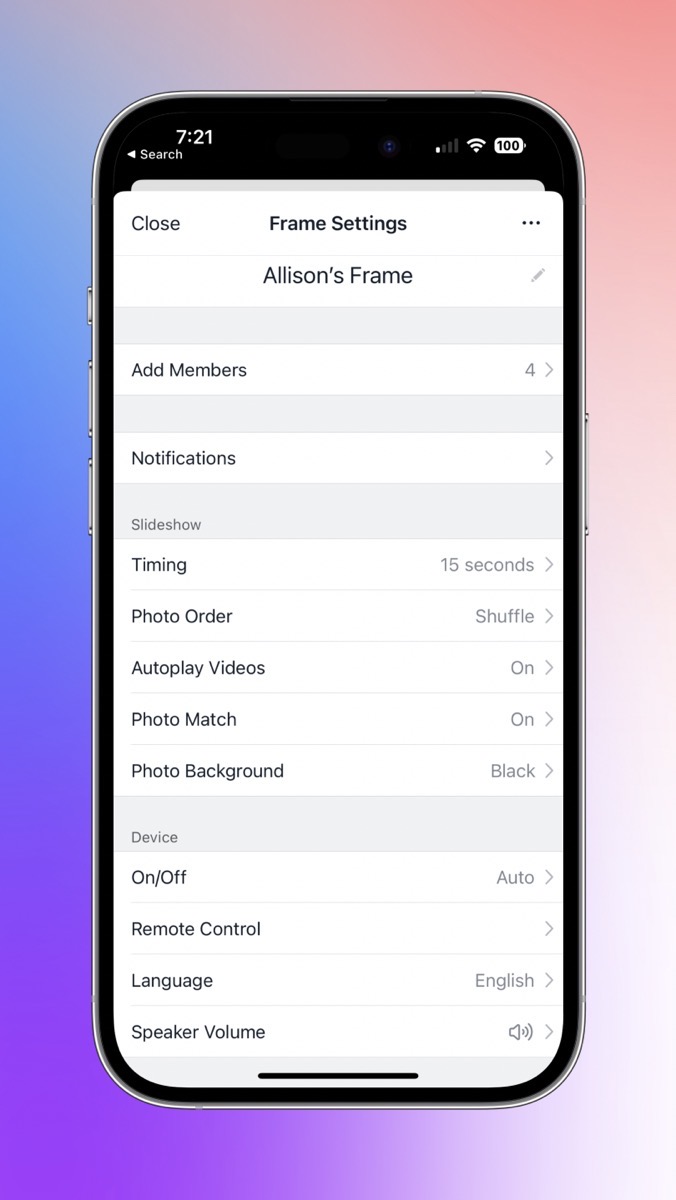This image features a black smartphone against a gradient background that transitions from blue on the left to slightly red on the right. The smartphone display shows a configuration screen with multiple settings, all written in black text. 

At the top left corner of the screen, there is an option labeled "Close Frame Settings" next to a menu icon. Below this, the screen displays the title "Alison's Frame" followed by the text "Add Members: 4," indicating that four members are currently added. Under the members section, it says "Notifications."

Below these options, additional settings and menus are organized:
- **Slideshow Menu Settings**:
  - **Timing**: Set to 15 seconds per photo.
  - **Photo Order**: Set to shuffle.
  - **Auto Play Videos**: Enabled.
  - **Photo Merge**: Enabled.
  - **Photo Background**: Set to black.

- **Device Settings**:
  - **On/Off**: Set to automatic.
  - **Remote Control**: Available.
  - **Language**: Set to English.
  - **Speaker Volume**: Set to full volume.

All the setting labels are aligned on the left side of the screen, with their corresponding values or options listed on the right. The overall background of the displayed settings is white, making the black text stand out clearly.